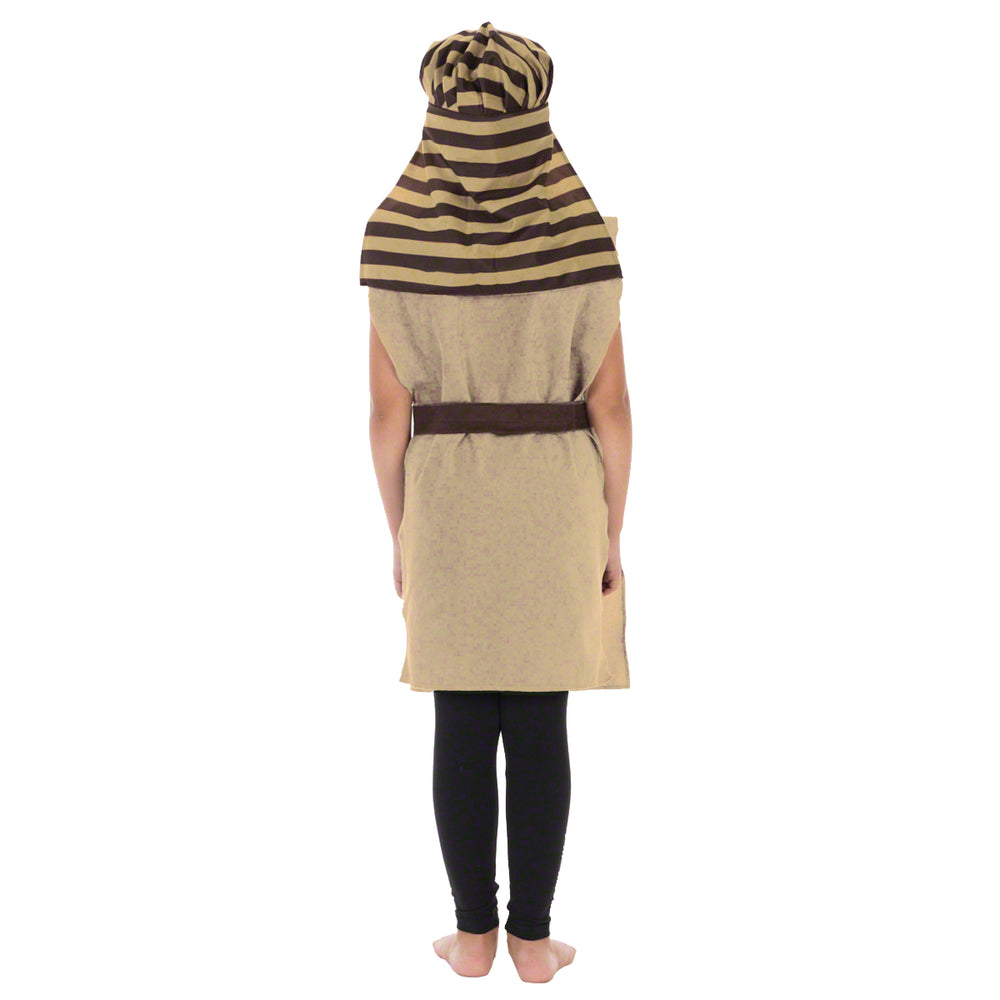This photograph captures the back of a person barefoot and wearing black tights, standing against a stark white backdrop. They are dressed in a sleeveless, knee-length, tan-colored jacket, cinched with a brown belt at the waist. The individual's position, hands tightly to their sides, emphasizes a simplistic yet striking attire hinting at an Egyptian pharaoh-inspired costume. Their head is adorned with a headdress made of mustard yellow and black stripes, which cascades down to their shoulders, enhancing the ancient, regal impression. Despite the costume's simplicity, perhaps symbolizing a less affluent pharaoh, the meticulous details—right down to the curves of their severely turned-in right ankle—paint a vivid, evocative image.